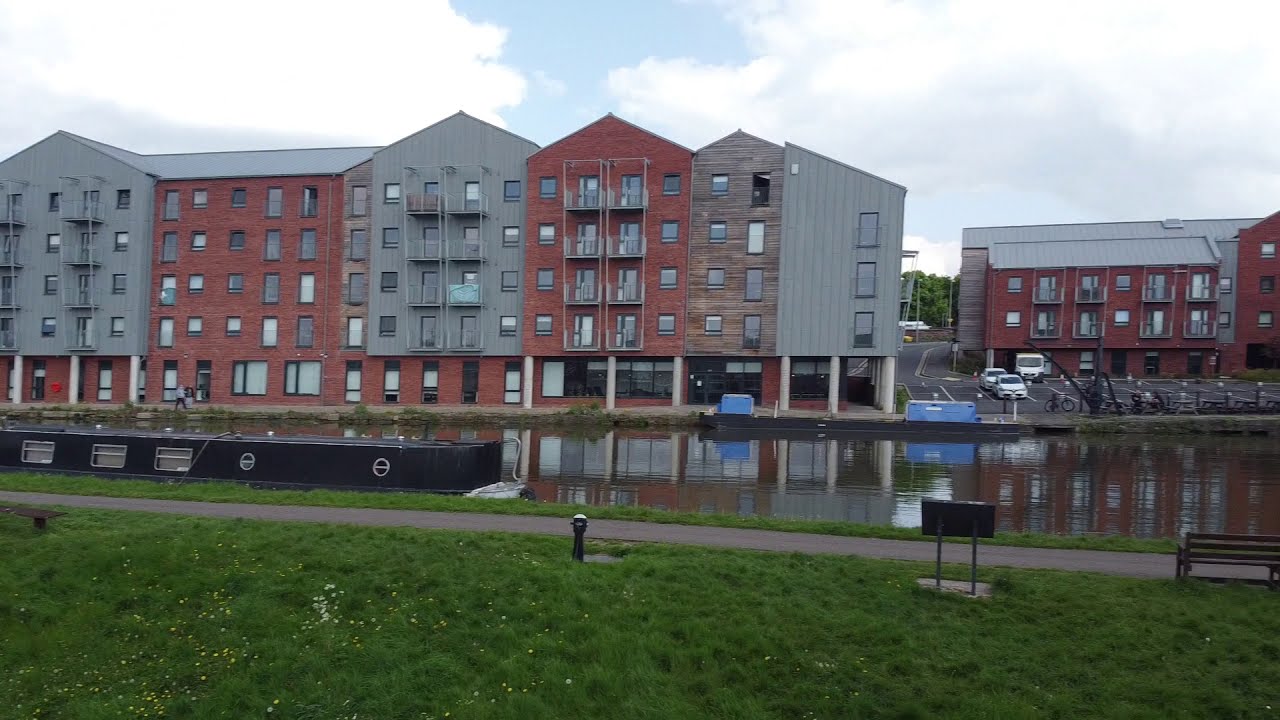This photograph depicts a multi-unit housing complex, possibly an apartment or condo community, set beyond a small body of water. In the foreground, a paved walkway is flanked by strips of green grass, sprinkled with flowers, and accented by a variety of objects including a potential barbecue stand, a standing object, and a bench to the far right. The water, which appears serene, acts as a central feature, adding a calming effect to the bustling housing scene beyond. Overlooking the water, two large, multi-story buildings rise, characterized by a distinct architecture featuring sections of gray tones and brick façades with V-shaped roofs. Each building includes terraces and vertical gray slats, indicating a mix of modern and traditional design elements. The complex is separated by a parking lot scattered with a few cars. To the left of the image, a dark-colored barge with three rectangular windows or vents floats on the water, adding a touch of industrial charm. The scene is set outdoors in the middle of the day under a blue sky dotted with clouds, enhancing the serene yet lively ambiance of the housing community.